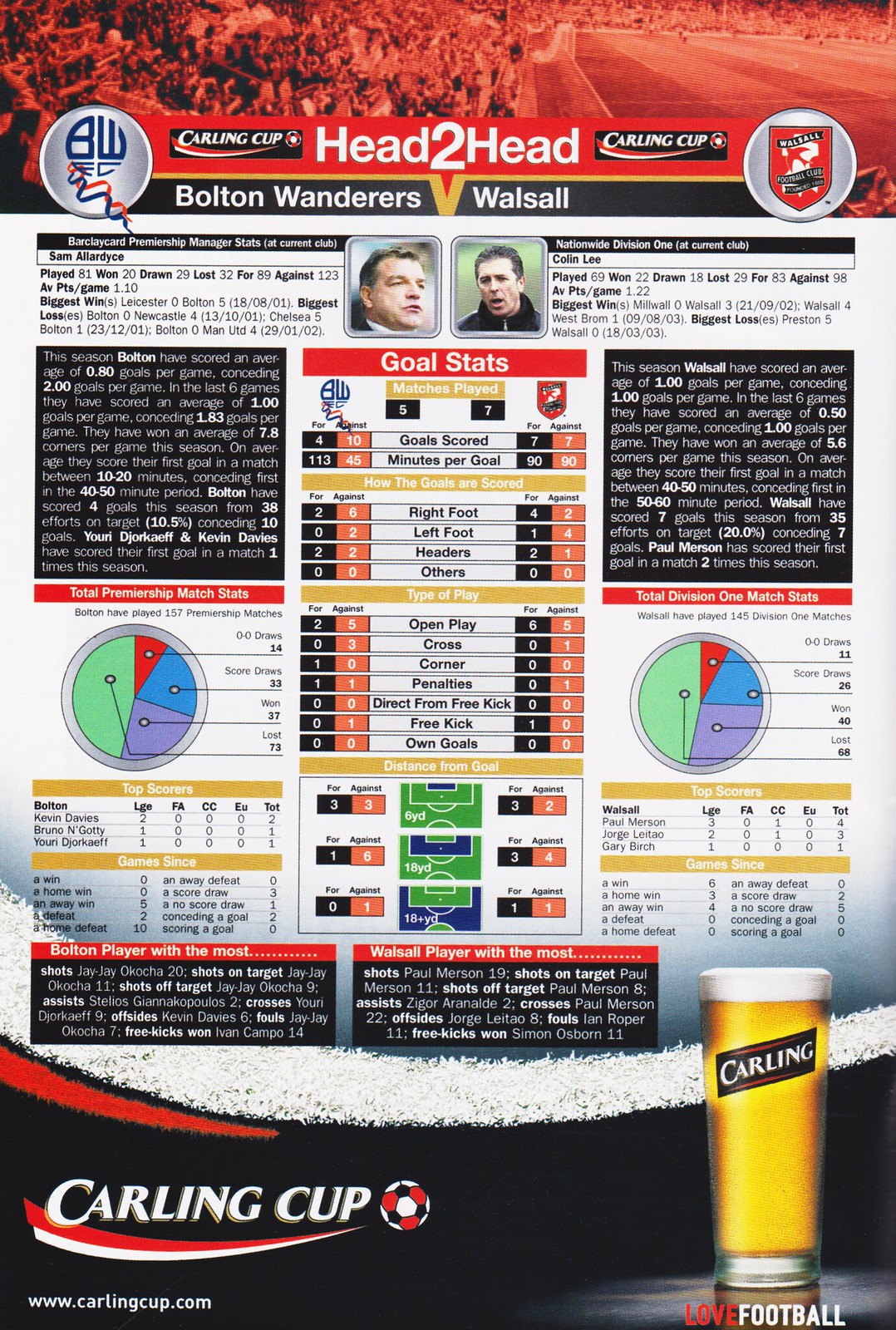The image showcases a detailed page from a magazine or program focusing on a curling cup, prominently titled "Carling Cup" at the top. Below, it features a "Head to Head" comparison between Bolton Wanderers and Walsall, set against a reddish backdrop depicting fans in the stands. Central to the page are images of two men, one in a white shirt and black jacket, the other in a black zip-up jacket. Beneath their photos, there are extensive goal statistics, including matches played, goals scored, and specifics such as right foot, left foot, headers, and more. Circular graphs displaying total Premiership match stats flank either side. At the bottom, in white letters against a black background, are the words "Carling Cup" and the website "www.carlingcup.com." To the right, there is a tall glass of yellow beer with a white foam top, branded with "Carling" in black and "love football" at the base.